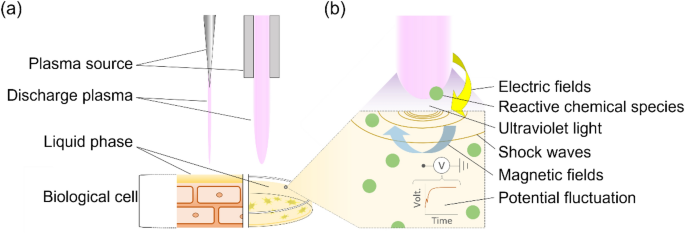The image is a detailed and colorful scientific diagram resembling a textbook drawing, depicting the process and effects of plasma discharge on a biological cell. To the left, it is labeled with black lowercase text identifying "plasma source," "discharge plasma," "liquid phase," and "biological cell." The plasma source is illustrated as an upside-down gray and white triangle connected to a purple line and two gray columns with a purple, upside-down rocket shape. Below this, a white box attaches to another box resembling bricks, which connects to a Petri dish containing green dots. Yellow and blue arrows emerge from this Petri dish, indicating various elements in the diagram.

Furthermore, the diagram includes a small B in a white circle with a black V, labeled "volt," connected by a red line to another element marked "time." To the right, detailed annotations and arrows point out electric fields, reactive chemical species, ultraviolet light, shockwaves, magnetic fields, and potential fluctuation. The diagram's components feature pink, green, and yellow with blue arrows, along with light brown, pink, and orange hues representing the biological cells. The entire diagram illustrates a comprehensive reaction mechanism, broken down into parts A and B, providing insight into the cellular responses to plasma exposure.